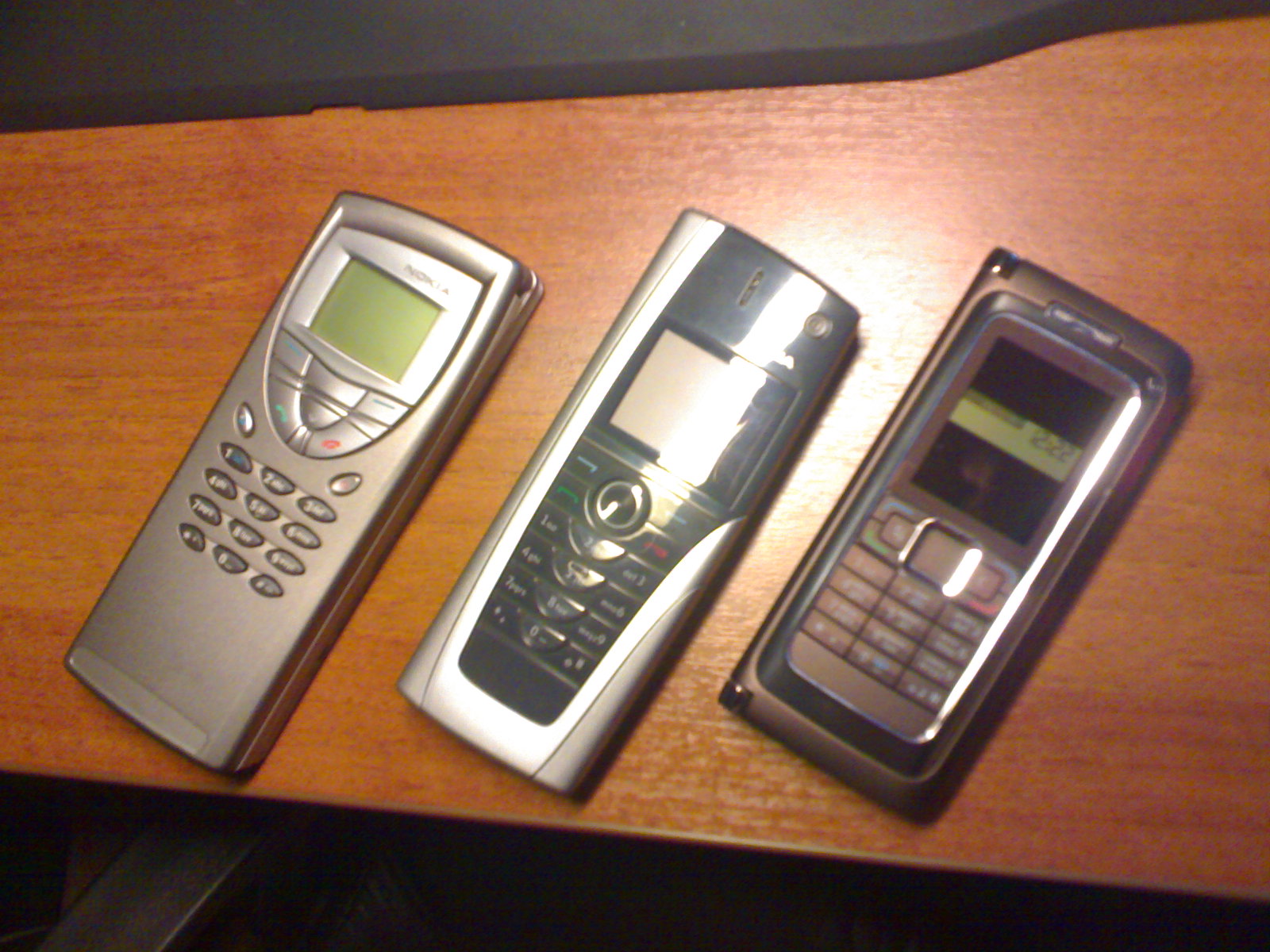The image features a slightly blurry photograph of three early 2000s candy bar style cell phones, arranged diagonally from the lower left to the upper right corner of the frame. Each phone has a small screen and physical push buttons, including green answer and red reject buttons. The phone on the left is a chromish silver Nokia with a recognizable brand logo, featuring a standard number pad and small screen. The middle phone, which caught the camera flash, is a silver and black device with similar physical buttons. The phone on the right is dark gray with larger, rectangular keys and a green-hued screen. All three phones are resting on an orange wood grain table, adding a vintage feel to the overall composition.